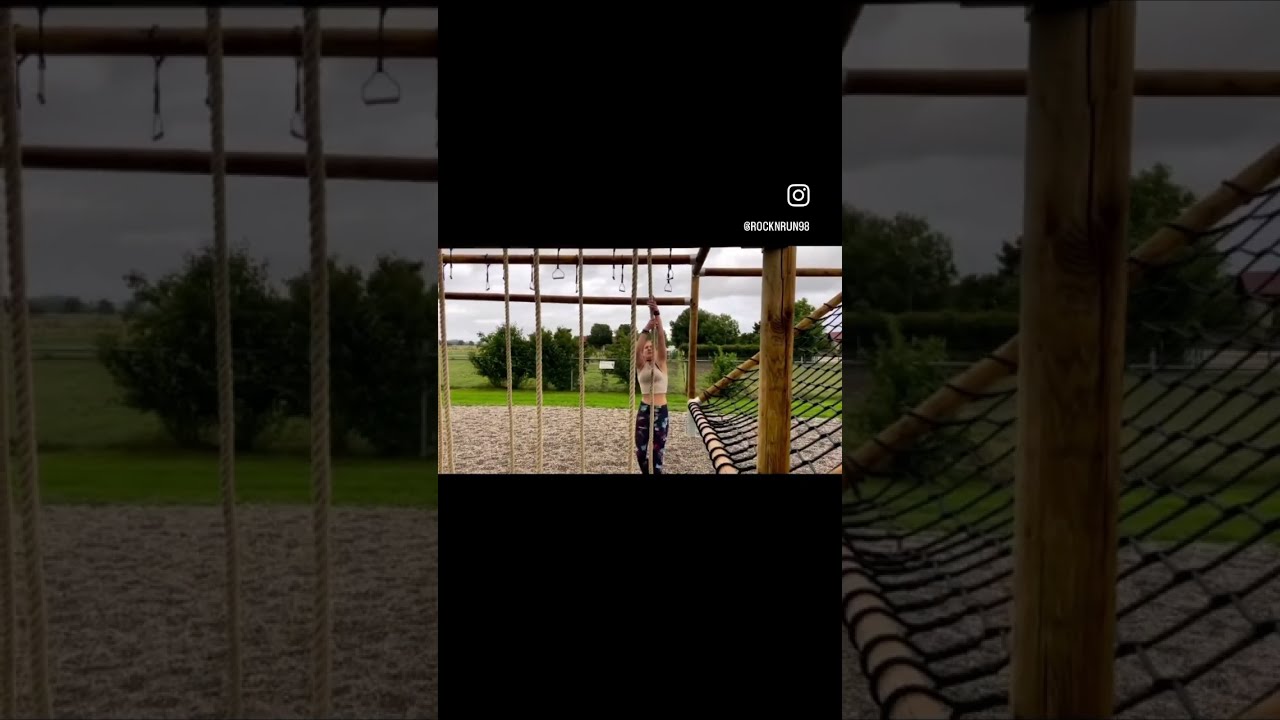The image is a color photograph framed in a portrait orientation with extended black panels at the top and bottom, centered within a larger horizontal frame where the base image is faded out on either side. The main focus is a horizontally rotated landscape-style picture, displaying an outdoor obstacle course. In the center, a young woman, dressed in black leggings with a distinct pattern and a gold crop top, reaches up towards handholds descending from an overhead rail. She appears to be navigating the obstacle course, which features various gym equipment including a climbing net on the right and several hanging ropes on the left. The background shows an overcast sky, a grassy field with low-growing trees, and shrubbery. Above the central image, there is an Instagram logo with the handle "Rock and Run 98" displayed in white text. The composition of the photograph exhibits a representational realism style.